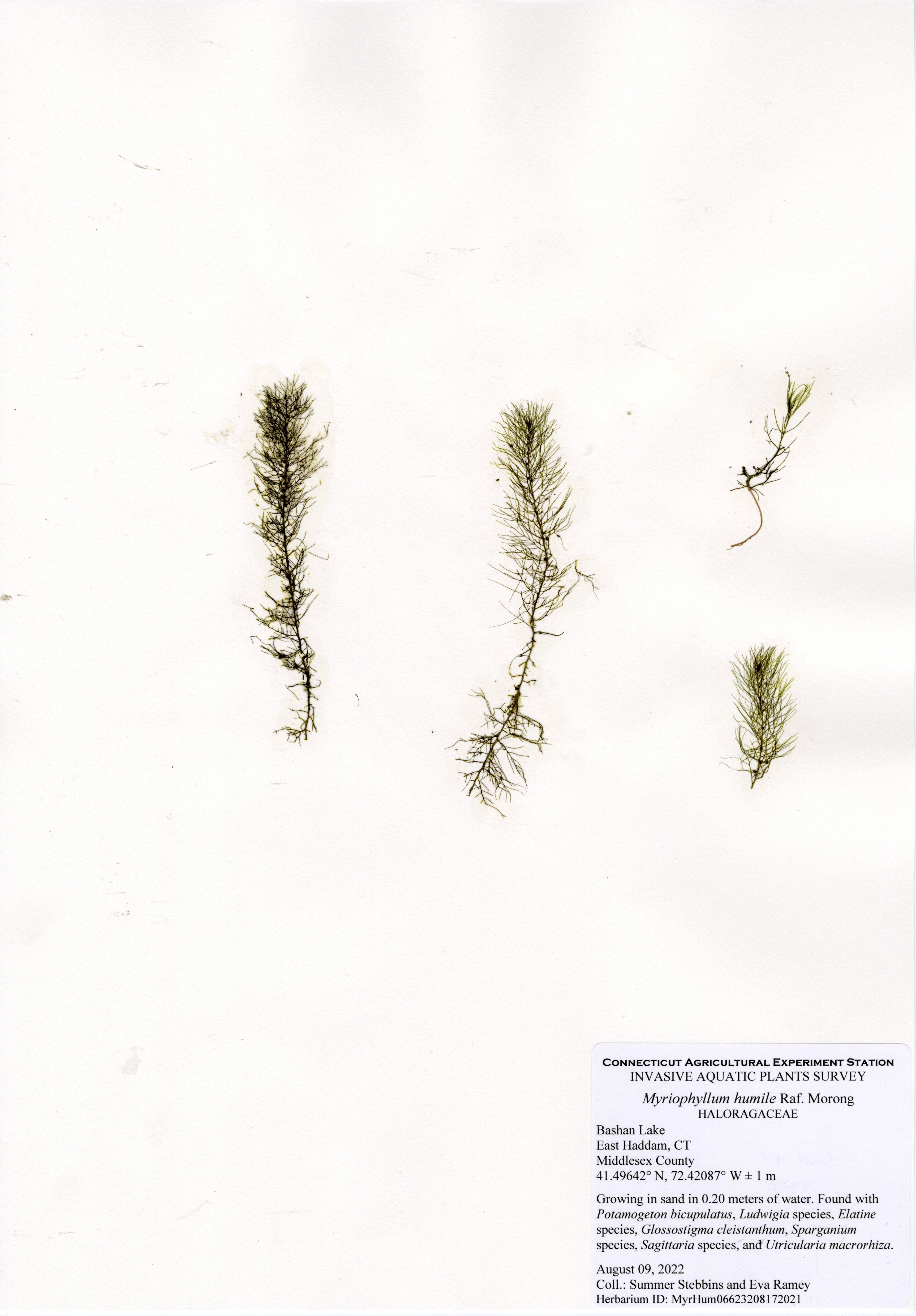This detailed photograph from the Connecticut Agricultural Experiment Station's Invasive Aquatic Plants Survey captures a collection of four aquatic plant species, including Myriophyllum humile, arranged centrally against a snowy white background. The photograph, taken at Basin Lake, East Haddam, Connecticut, Middlesex County, documents plants grown in sand and 0.20 meters of water, found alongside other species such as Potamogeton bicupulatus, Ludwigia, Elytine, Glossostigma, Clastanthium, Sperganium, Sagittaria, and Atricularia macrohyza. The plants exhibit shades of green and dark green, contrasting with the predominantly black, white, and gray surroundings. The position of the plants spans from the middle to the right of the frame, while a descriptive label providing further context and geographic coordinates (41.49624° N, 72.42087° W) is located in the bottom left corner. This image, identified under Herbarium ID MYRHUM 06623208172021 and collected by Summer Stebbins and Eva Ramey on August 9th, 2022, offers a meticulous representation of the species present in the surveyed aquatic environment.